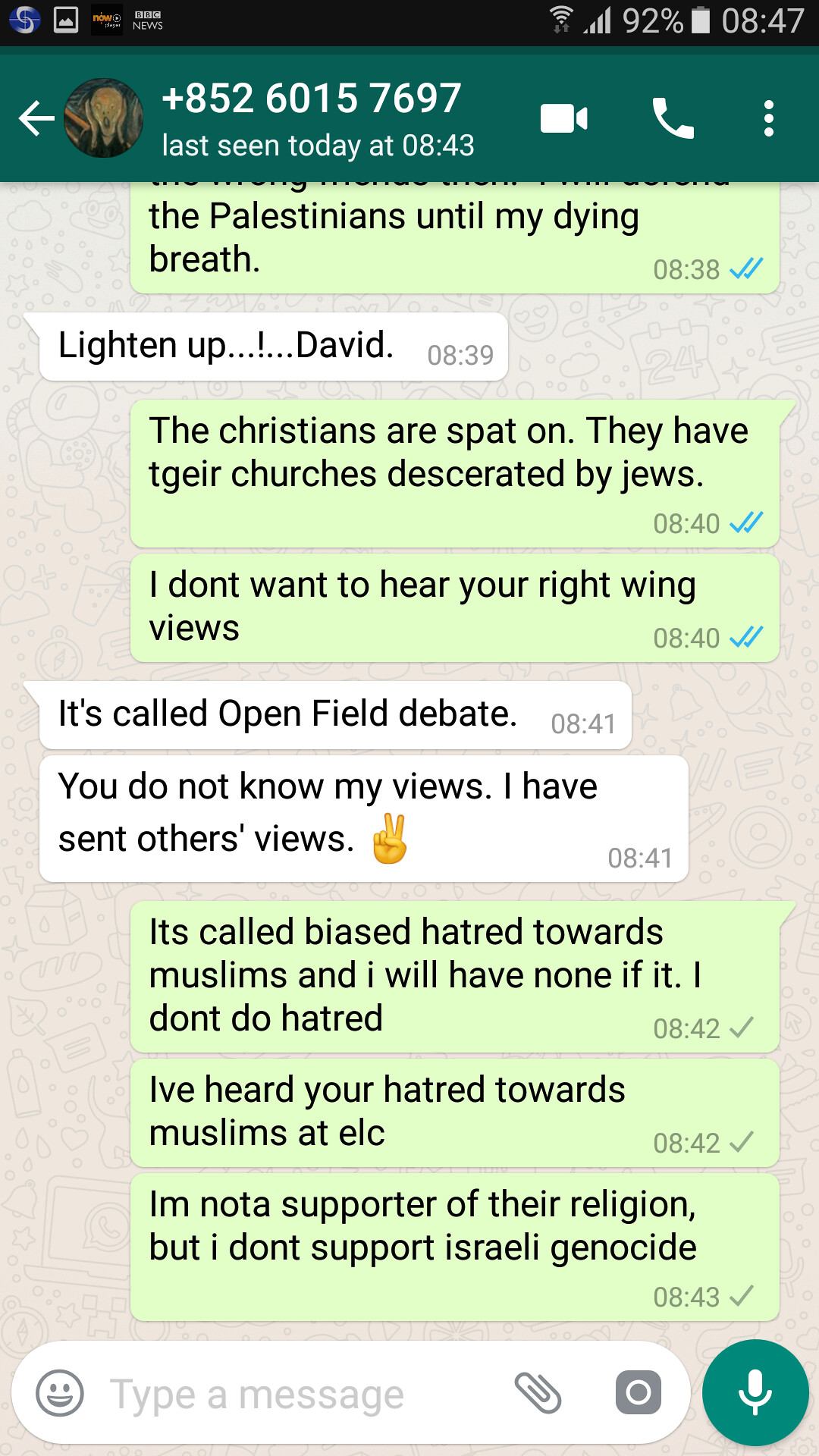The image shows a detailed screenshot of a text message conversation on a phone. The header of the conversation includes the phone number, "852-601-57697," and an avatar featuring Edvard Munch's "The Scream." The status bar at the top indicates the time is 8:47, with the phone being charged at 92% and connected to a full-strength WiFi signal. 

The header of the messaging app displays "last seen today at 8:43," and there are icons for a camera, a phone, and three dots indicating further options. The conversation is a heated debate on sensitive topics surrounding Israel and Palestine, and interactions between Christians and Jews. Incoming messages are shown in light green and outgoing messages in white. Text exchanges include statements such as "lighten up David" and counterpoints like, "The Christians are spat on. They have their churches desecrated by Jews." Further exchanges become more intense, with messages stating, "I don't want to hear your right-wing views" and "It's called biased hatred toward Muslims, and I will have none of it."

At the bottom of the screenshot is a text input field labeled "type a message," accompanied by icons for attaching files, photos, and recording audio. The phone shows a background in a gray hue, complementing the stark and contentious nature of the conversation displayed.